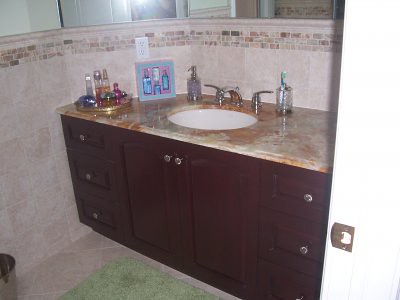This indoor photograph showcases a meticulously designed bathroom. At its center is a singular white porcelain sink embedded in a countertop made of marble that exhibits an array of colors including reddish-brown, light gray, and off-white. Complementing the elegant sink, the faucet and handles are crafted from silver metal. The walls are adorned with softly colored, dusty rose pink tiles, creating a warm and inviting atmosphere. Mirrors, curving gracefully around the walls above the tiles, reflect the entirety of the room. The floor is made of tiles matching those on the walls, maintaining a consistent aesthetic. 

Directly in front of the sink lies a plush green carpeted-style rug, adding a touch of comfort underfoot. Dark wooden cabinets with silver round handles sit beneath the sink, all neatly closed, providing storage and enhancing the room’s sophistication. On the right side of the sink, an empty soap dispenser sits, while on the left, another soap dispenser resides next to a stylish collection of bottles. This ensemble appears to be a curated set of perfumes and bath products, adding both functionality and a hint of luxury to the bathroom’s décor.